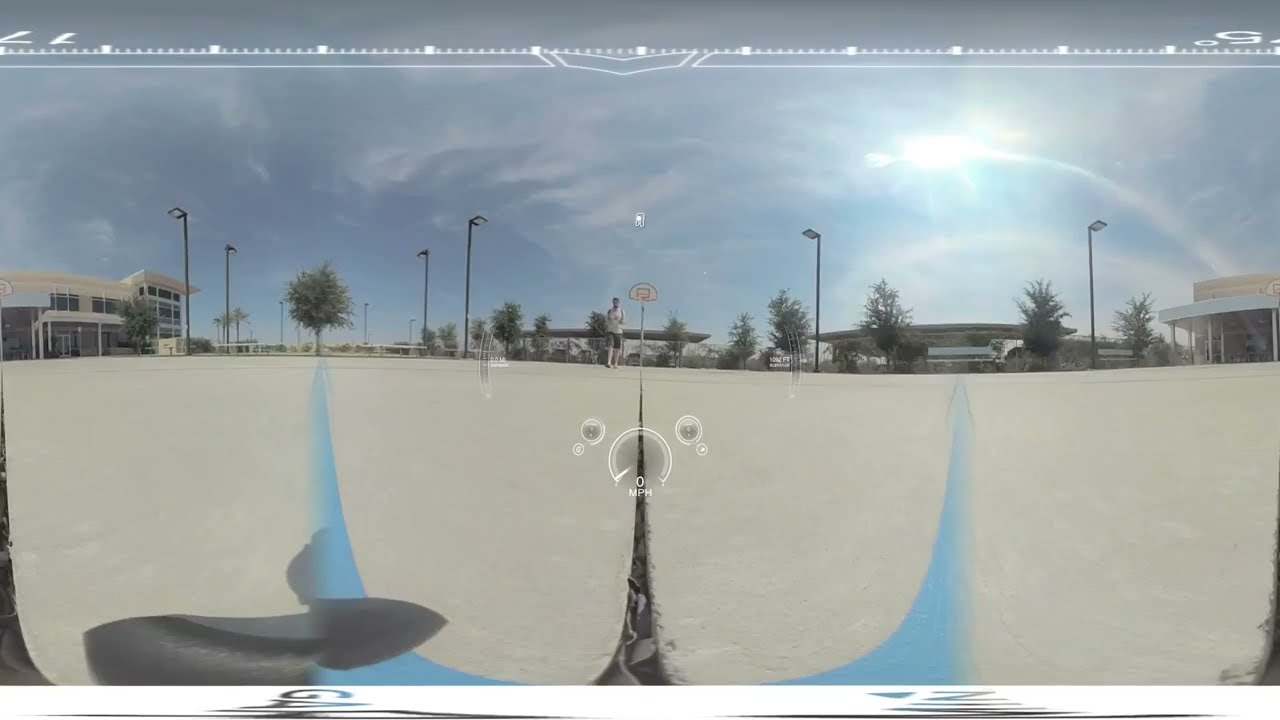The image presents a distorted, fisheye view, likely from a video game, creating a circular effect on straight lines. Dominating the center of the image is a white circular gauge which reads zero MPH, with a dial pointing downwards. Above the central gauge, which might be part of a heads-up display, there are additional indicators, including an upside-down number 77 on the left and an upside-down 5° on the right. The scene depicted is a basketball court made of gray or light tan cement. Directly ahead, a basketball hoop is visible, and a blue streak runs from the left side of the court, curves, and ascends towards the right, intersected by a black line pointing towards the hoop.

To the left of the hoop stands a man dressed in a white t-shirt and gray or dark shorts, walking forward. Behind him are several buildings. The central building appears to be a covered structure with a flat metal roof and is surrounded by trees and streetlights—around nine of them, tall with square lights facing downward. On the far left is a cream-colored building with a glass front. To the far right, another cream-colored building features a balcony with a white covering supported by white poles. It’s a sunny day with visible clouds in the sky, and the upper right corner of the image is particularly bright due to the sun’s light. The scene gives an impression of a sparse background, suggestive of a school or institutional environment.